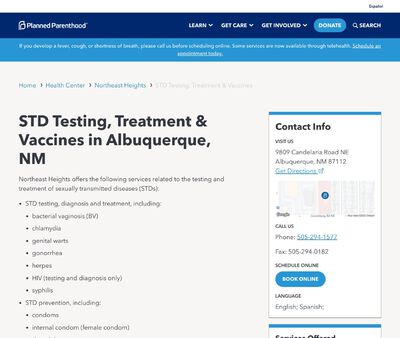The image features a detailed informational flyer for the Northwest Heights Health Center in Albuquerque, New Mexico. 

**Header:**
- A white bar at the top contains the word "Español" in black text on the right-hand side. 
- Beneath this, a blue background spans the width of the flyer. On the left, "Planter" is written in white text. On the right, phrases such as "Learn," "Get Cared," and "Get Involved" are listed, along with a blue button labeled "Donate" in white text. A search option is also present on the right side. 

**Main Body:**
- In the next section with a blue background and white text, there is text that is partially illegible, but the last four words are underlined. 
- Following that, the white background section includes clear, black text stating: "It's Home, Health Center, Northwest Heights." A few elements in gray text are present here but are difficult to make out. 

**Medical Services:**
- The flyer lists a comprehensive range of services related to sexually transmitted diseases (STDs). These include:
  - **Testing and Treatment for:**
    - Bacterial Vaginitis (BV)
    - Chlamydia
    - Genital Warts
    - Gonorrhea
    - Herpes
    - HIV (Testing and Diagnosis Only)
    - Syphilis
  - **STD Prevention:**
    - Condoms
    - Internal Condoms (Female Condoms)
 
**Contact Information:**
- The right-hand side of the flyer is divided into blue sections at the top and bottom, with the central part in white. 
- "Contact Info" in black text outlines:
  - "Visit Us" at 9809-something, Northeast, Albuquerque, New Mexico.
  - A phone number is provided, and there is an option to book online.

**Footer:**
- "STD Testing, Treatment and Vaccines, Albuquerque MD, New Mexico" is prominently displayed.

The detailed layout and comprehensive service information make this flyer a valuable resource for individuals seeking STD-related healthcare services at the Northwest Heights Health Center.